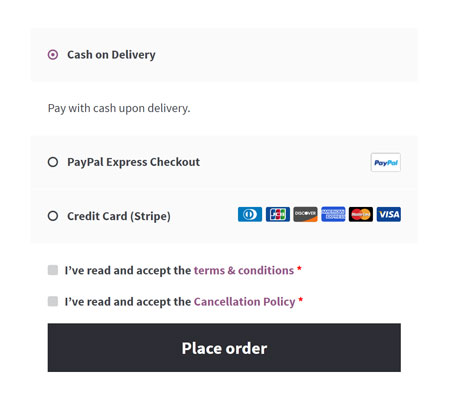At the top of the image, there is a light gray rectangle. Below it, a purple circle is present with a purple inner element that reads "Cash on Delivery." Adjacent to this circle is a white rectangle containing the text "Pay with cash upon delivery."

Moving down, there's another light gray rectangle that features a black-outlined circle labeled "PayPal Express Checkout." To its right, a gray outlined rectangle displays the word "PayPal" in a combination of dark blue and light blue.

Further down, another gray outlined rectangle has a black-outlined circle that says "Credit Card" and includes the text "Stripe." To the right of this, various credit card logos are shown, including recognizable ones like American Express, MasterCard, Visa, and Discover, as well as two unidentified logos.

Next, there is a gray square containing the text "I've read and accepted the terms and conditions" with "terms and conditions" highlighted in purple and a red star next to it. Below this, another gray square states "I've read and accept the cancellation policy," with "cancellation policy" also in purple and accompanied by a red star.

At the bottom of the image, a black rectangle is prominently displayed with the words "Place Order" in white font.